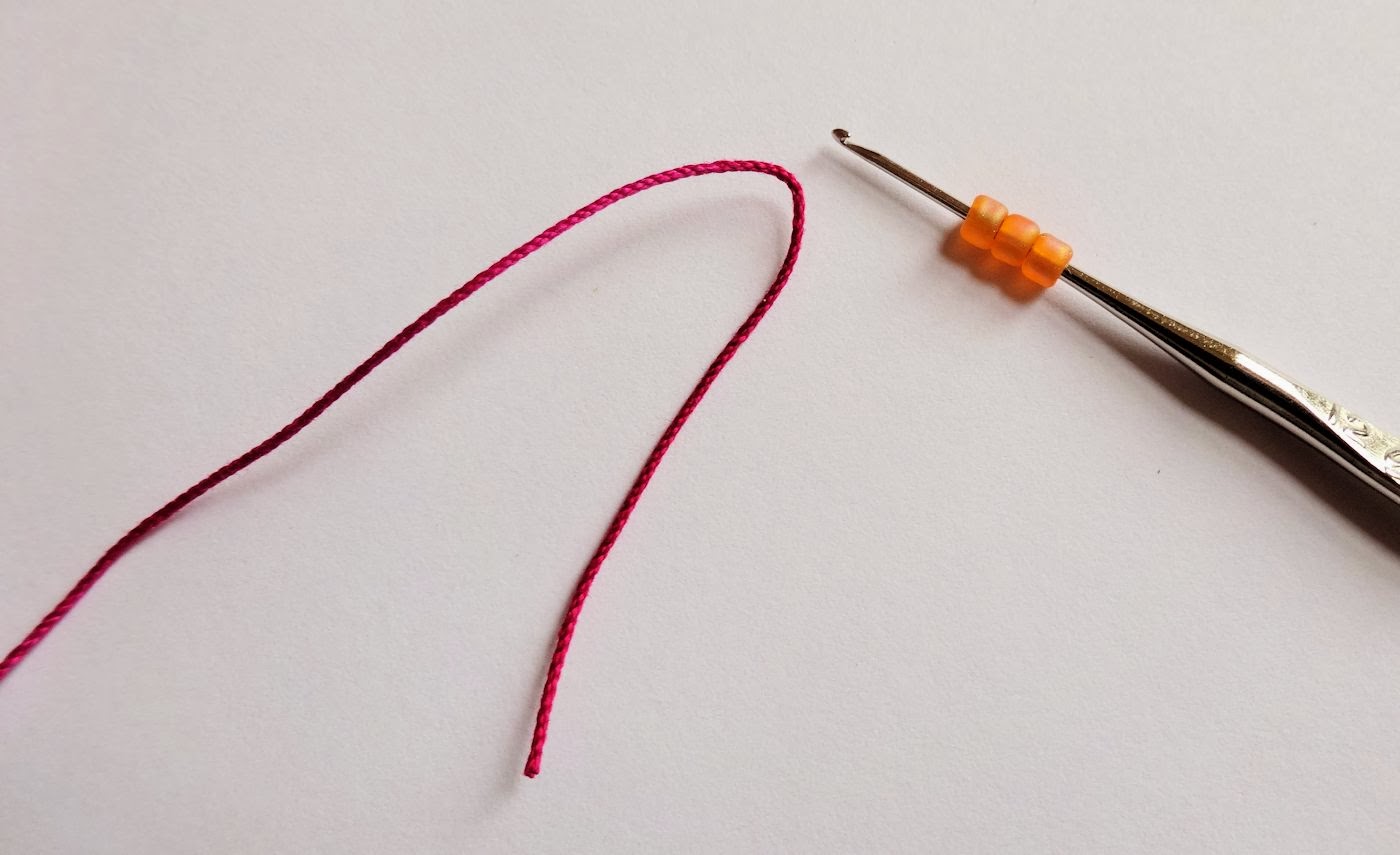The image exhibits a simple and precise scene set against a white background. A vivid magenta string, positioned diagonally, curves gracefully up and then back down with a clean-cut end. To the right of the string, a silver-colored crochet hook enters the composition diagonally, partially visible with three orange, circular beads threaded onto its pointed part. The beads are situated about halfway down the hook, which thickens toward the bottom, preventing the beads from sliding further. The crochet hook also features a flat section on its side, marked with the number "12." The overall lighting comes from the upper right, casting slight shadows and highlighting the vibrant colors and metallic sheen of the hook.